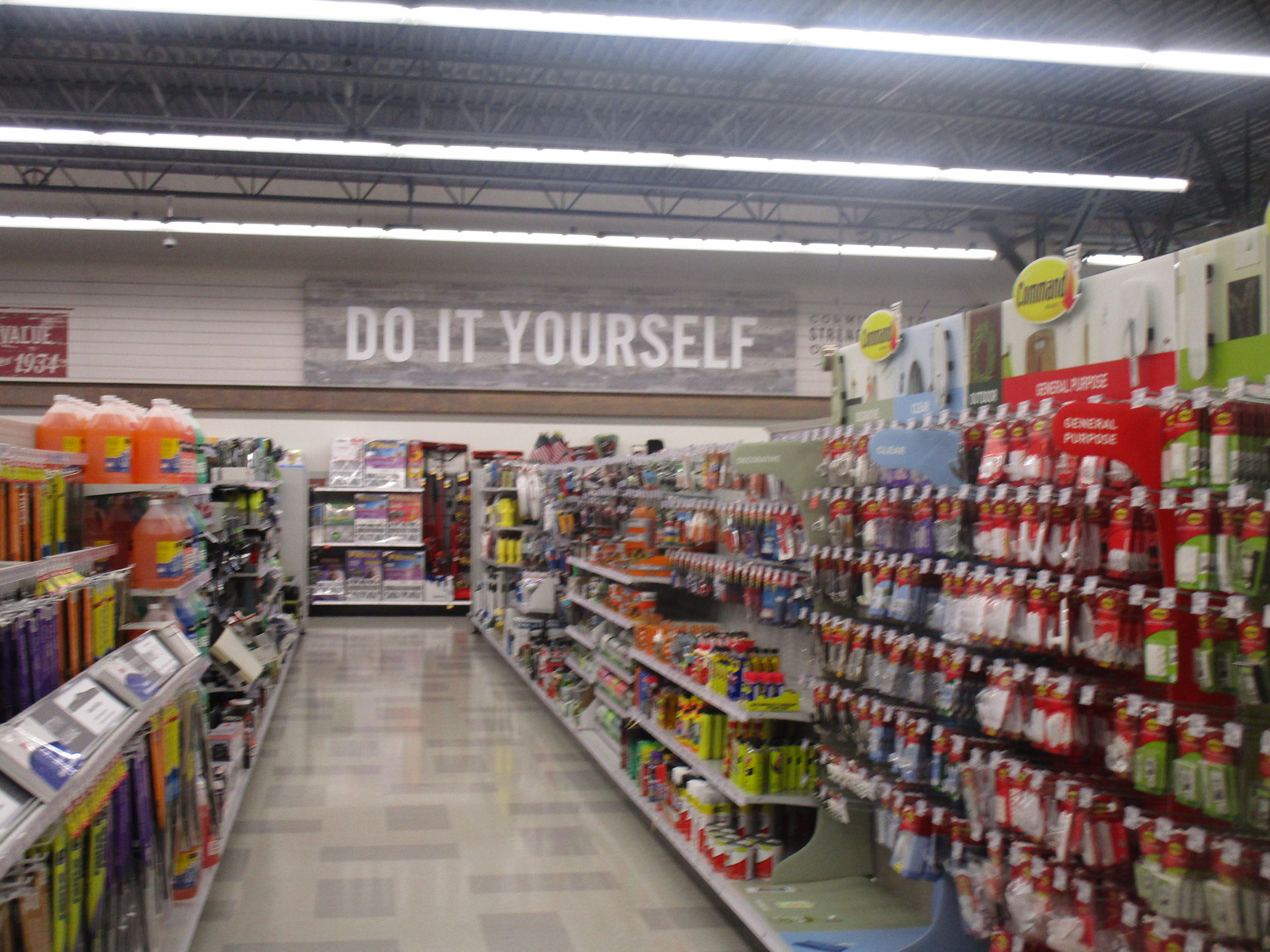This is a detailed color photograph taken inside a hardware store, specifically in an aisle dedicated to do-it-yourself items. The floor is covered in gray and tan linoleum tiles, and the walls are made of white brick. On the back wall, high up, there's a gray sign with white capital letters reading "DO IT YOURSELF." The ceiling is painted black and features black metal poles with horizontal fluorescent lighting, ensuring the aisle is brightly lit.

On the left side of the aisle, various products are neatly organized. These include windshield wiper blades, jugs of coolant and other fluids in vivid orange, green, and blue colors, visible with yellow labels. On the right side, there are numerous 3M hooks, sticky wall hangers, and adhesive mounts hanging from the shelves. Bright reds, greens, oranges, yellows, and blues dominate the scene, adding to the visual appeal and highlighting the diversity of items available. Price tags are visible everywhere, further emphasizing the retail environment.